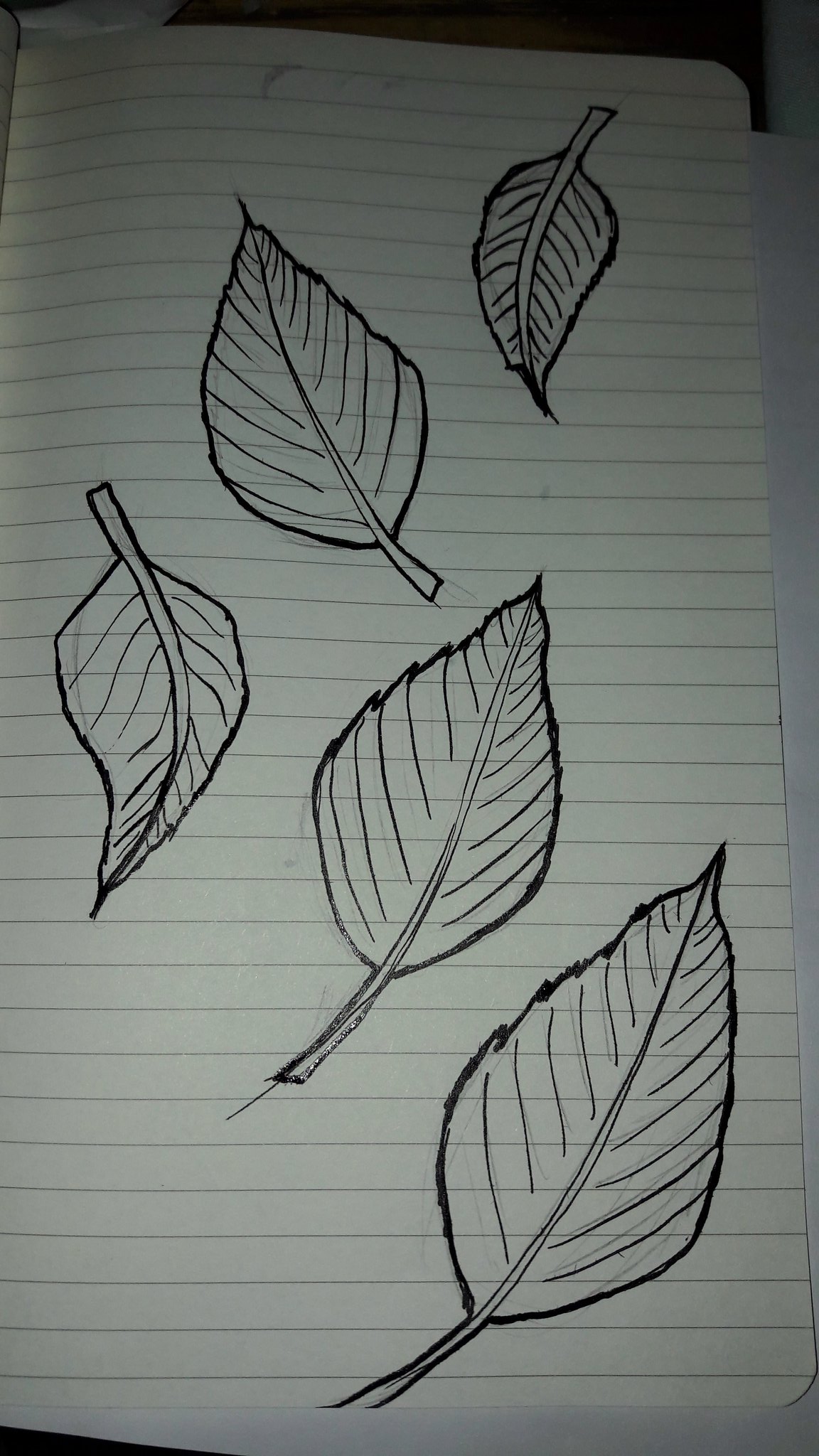This captivating image showcases a piece of fine, white-lined paper adorned with intricate black pen drawings of five leaves. Each leaf, though varying slightly in size, exhibits a consistent artistic style, creating a harmonious visual theme. Delicate lines intricately trace the veins of the leaves, converging towards the pronounced midrib that extends from the top of each leaf to just beyond its base, where the lines appear to be cut off. The composition places two leaves in the bottom right corner and three leaves in the upper left corner, balancing the arrangement elegantly. The deliberate detailing and thoughtful placement of each leaf against the simplicity of the lined paper evoke a sense of natural beauty interlaced with meticulous craftsmanship.